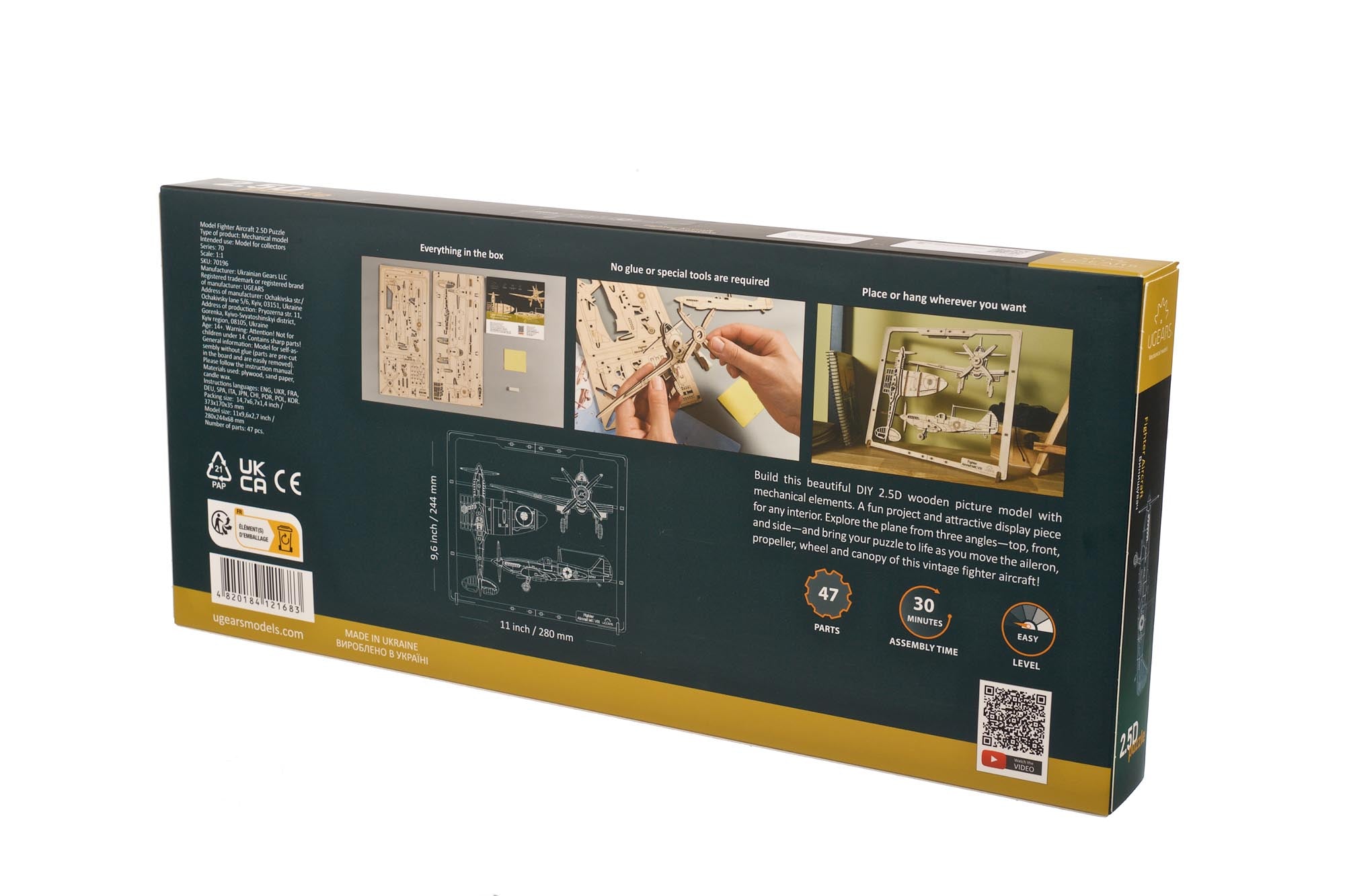This horizontal, isometric-view photograph showcases the back of a product box, potentially for a kit of a World War II plane assembly set. The box itself is dark gray with gold corners and a gold strip running across the bottom edge. A notable feature is the upper text detailing the product’s specifications, which includes 47 parts and an average assembly time of 30 minutes, highlighting its ease of use. On the lower right corner, a UR code invites scanning for additional information. Nearby, a barcode and several approval marks from various agencies are visible.

Prominently, the back is organized with three photographs that illustrate the assembly process: 
1. The first photo depicts two flat boards with pre-cut pieces alongside an instruction booklet.
2. In the middle photo, two hands are shown actively working on assembling the kit.
3. The final photo likely shows the finished product or a detailed diagram displaying multiple views of the plane from different angles.

Overall, the detailed descriptions and imagery aim to guide the user through the assembly process while promoting the product's simplicity and completeness.